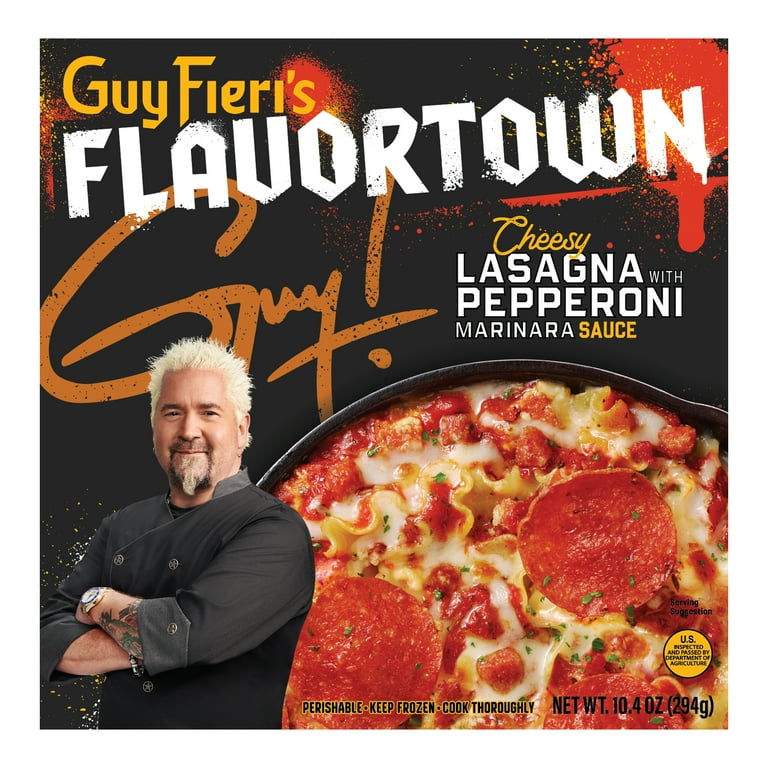The image showcases a box of frozen Italian food labeled "Guy Fieri’s Flavortown Cheesy Lasagna with Pepperoni Marinara Sauce." The box features a striking black background accented with red designs. Prominently displayed in the top left is a photograph of Guy Fieri from the waist up. He is smiling at the camera with his arms crossed, wearing a black shirt, a wristwatch on his left wrist, and a bracelet on his right. His signature spiky white hair and a goatee complete his iconic look.

Beside Guy Fieri’s image, the product name is boldly written: "Guy Fieri’s" in gold and "Flavortown" in white, utilizing a vintage font. Directly beneath this, it describes the dish as "Cheesy Lasagna with Pepperoni Marinara Sauce." 

The right side of the package features a close-up photo of the lasagna, showing layers of pasta, marinara sauce, melted cheese, and pepperoni slices. At the bottom of the box, the necessary handling instructions are clearly printed: "Perishable, keep frozen, cook thoroughly," along with the net weight of 10.4 ounces (294 grams). An autograph from Guy Fieri, appearing in gold cursive, adds a personal touch to the design.